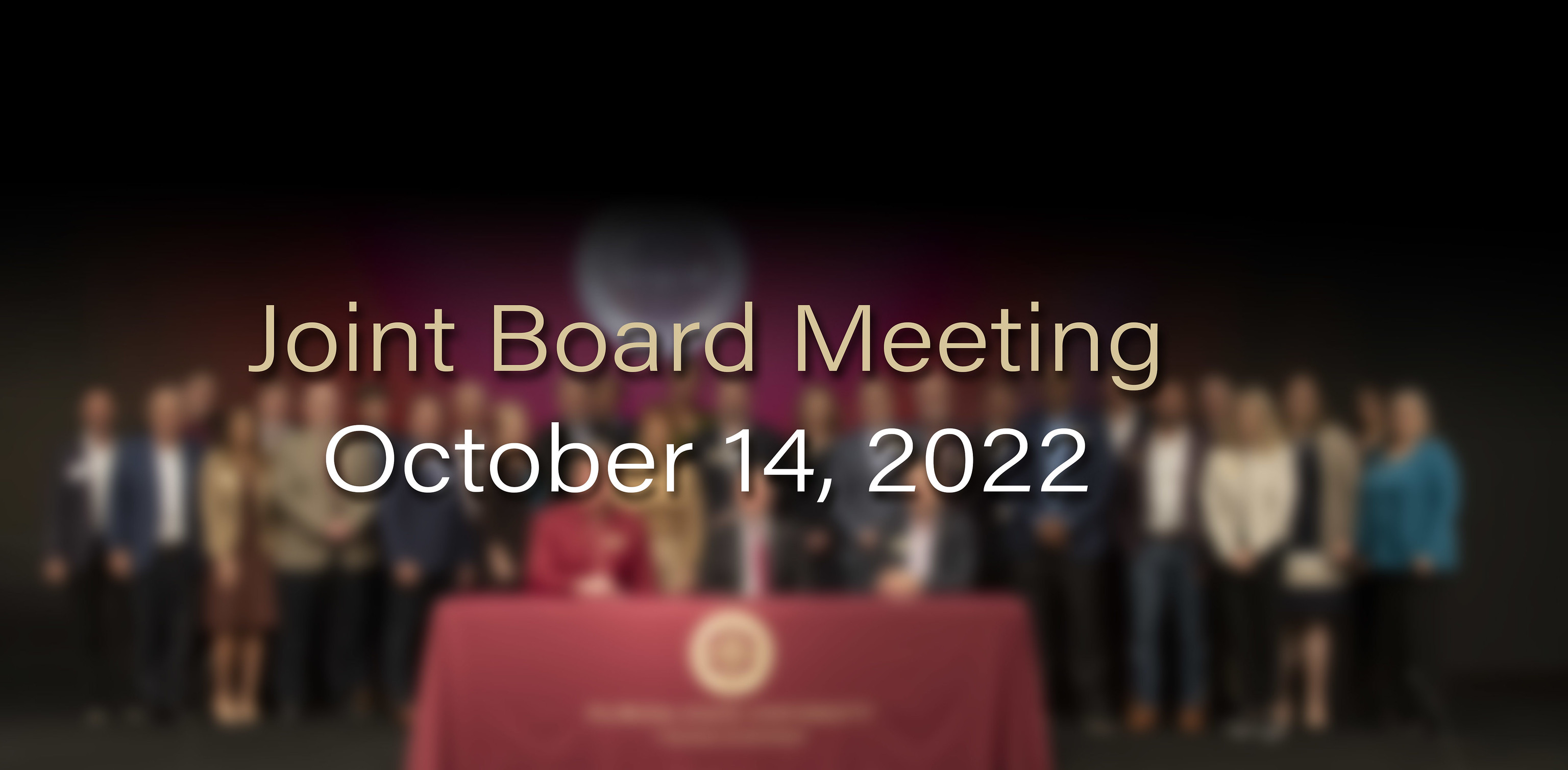The image captures a promotional scene for an event, specifically a "Joint Board Meeting" held on October 14, 2022, as indicated by gold and white text overlaying the image. The setting features a blurred background where several people, both men and women dressed in business attire, stand against a wall with indistinct details. Noteworthy, on the right side of the image, is a woman in a blue top with blonde hair, her hands resting by her side. In the foreground, a long table draped with a vibrant red cloth adorned with a gold emblem hosts three seated individuals. They are presumably participating in the meeting and dressed formally, possibly with microphones on the table, hinting at their roles in the event. The overall image is shadowy with a black background, emphasizing the professional and formal atmosphere of the meeting.